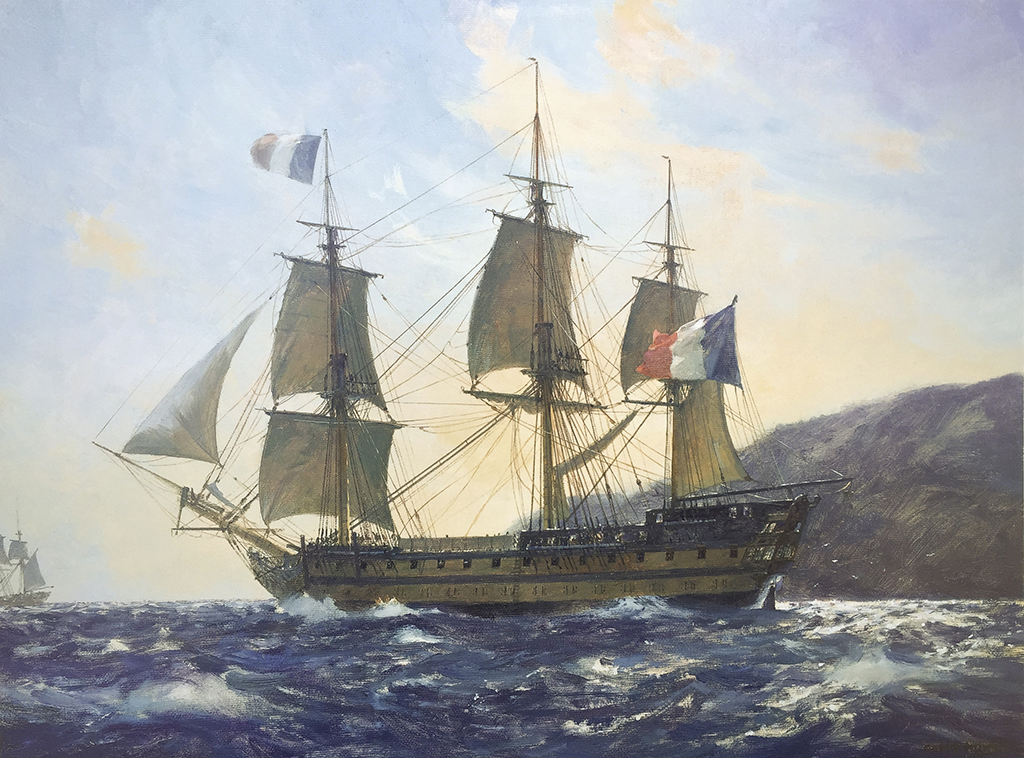The image depicts a detailed painting of an ancient sailing vessel prominently featuring the tricolor flag of France on both the rear and front mast. The light brown and black ship is navigating choppy, dark blue waters, with its sails full and the wind animating its flags. In the background, on the left side, there’s another smaller sailing vessel. The scene is set outdoors under a bright blue sky dotted with patches of white clouds. The right side of the image showcases a coastline with a dark brown hill. The waves, sun high in the sky, and the overall bright and clear lighting bring the seascape to life, highlighting the ship’s many broadside cannons and its journey to the sea.